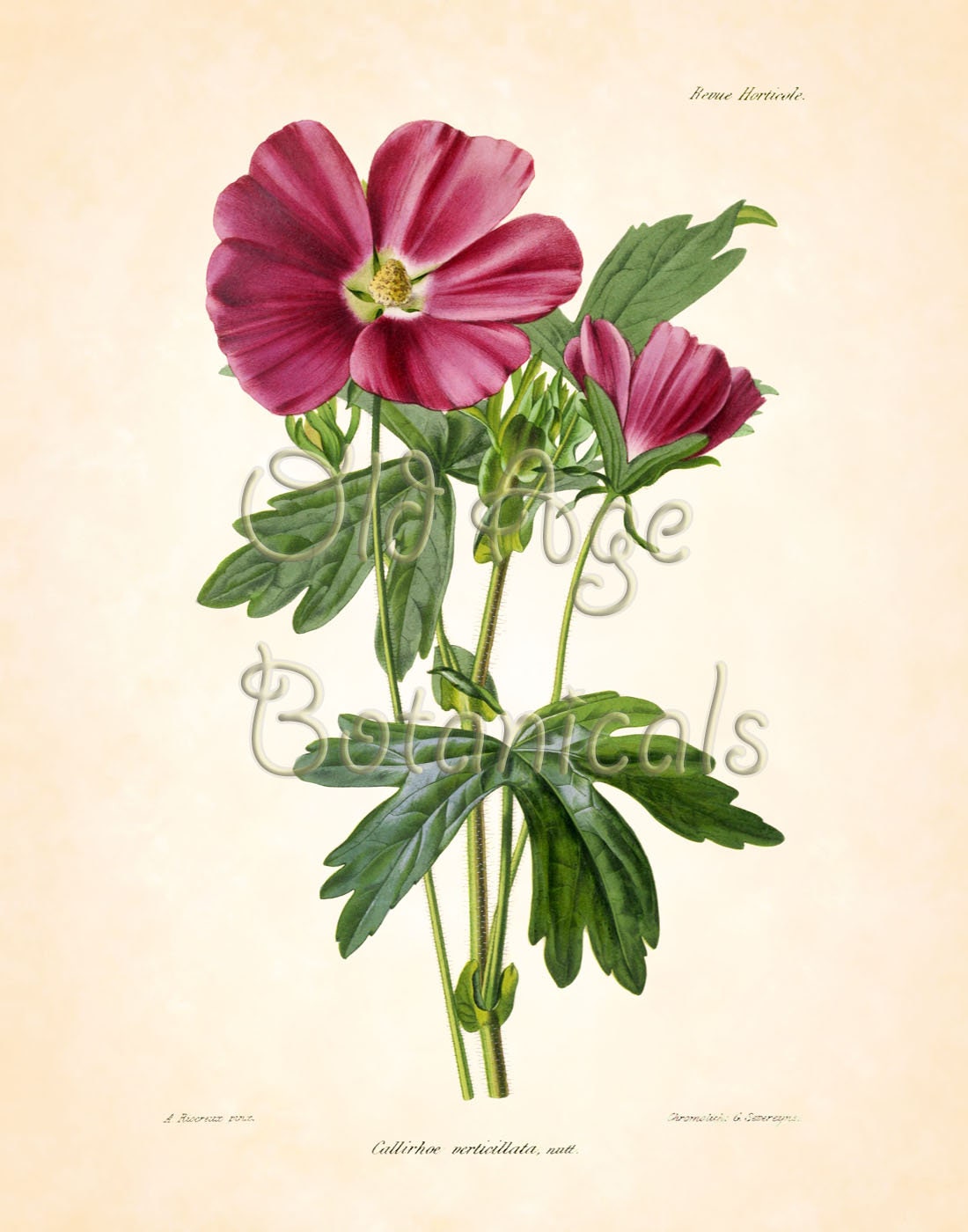This is a detailed, hand-painted botanical illustration of two pinkish-red flowers, possibly roses. The primary flower on the left is fully bloomed with its delicate petals spread open, showcasing a yellow center. The accompanying flower on the right is partially closed, indicating it is in the early stages of blooming. Both flowers have vibrant green stems adorned with lush green leaves clustered towards the top and smaller leaves at the base. Above the illustration, the name "REVUE HORTICOLE" is inscribed, likely indicating the publication or artist's signature. The background of the image is a bright, parchment-like color, emphasizing the floral details. At the bottom, the scientific name "Calorimorticoata" is faintly visible, albeit slightly out of focus, adding to the botanical and scientific authenticity of the piece. The caption "Old Foggy Botanicals" is centrally placed, reinforcing the traditional, scientific nature of the illustration.